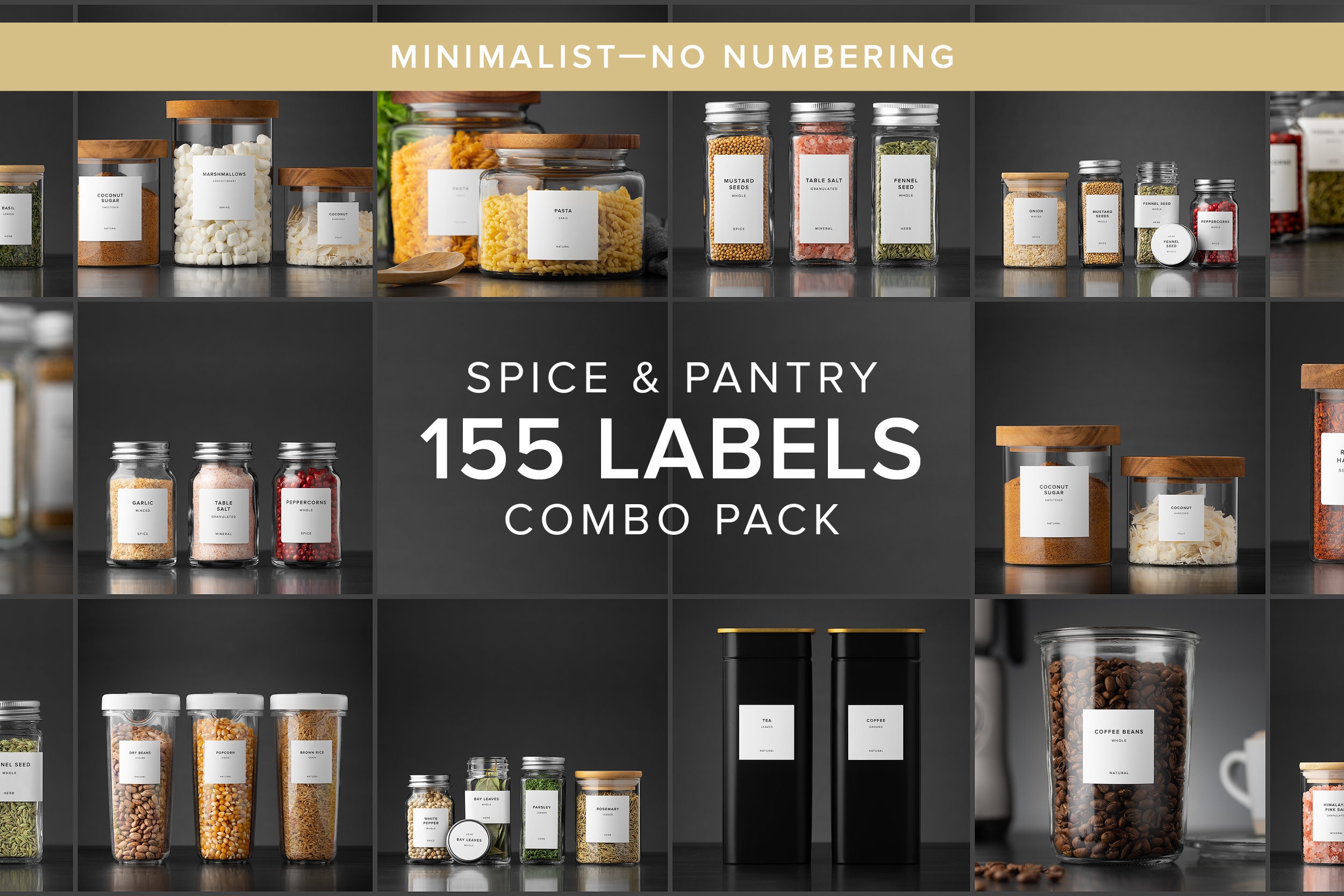This advertisement showcases a comprehensive "Spice and Pantry, 155 Labels Combo Pack" for organizing kitchen essentials. The ad is designed with a three-by-five grid of photographs, each featuring a variety of spice jars and pantry containers with clear white labels bearing black text, though the specific label text is not legible. The jars are filled with various pantry items such as spices, pink salt, pasta, and coffee beans. Centered in the image is a prominent black square with white text announcing the label combo pack. At the top of the advertisement, a tan-colored banner with the words "Minimalist, no numbering" emphasizes the label design philosophy. The containers displayed range from clear glass jars with silver, plastic, and brown wooden lids to solid black containers with gold lids, each contributing to a sleek and organized kitchen aesthetic against a dark gray background.